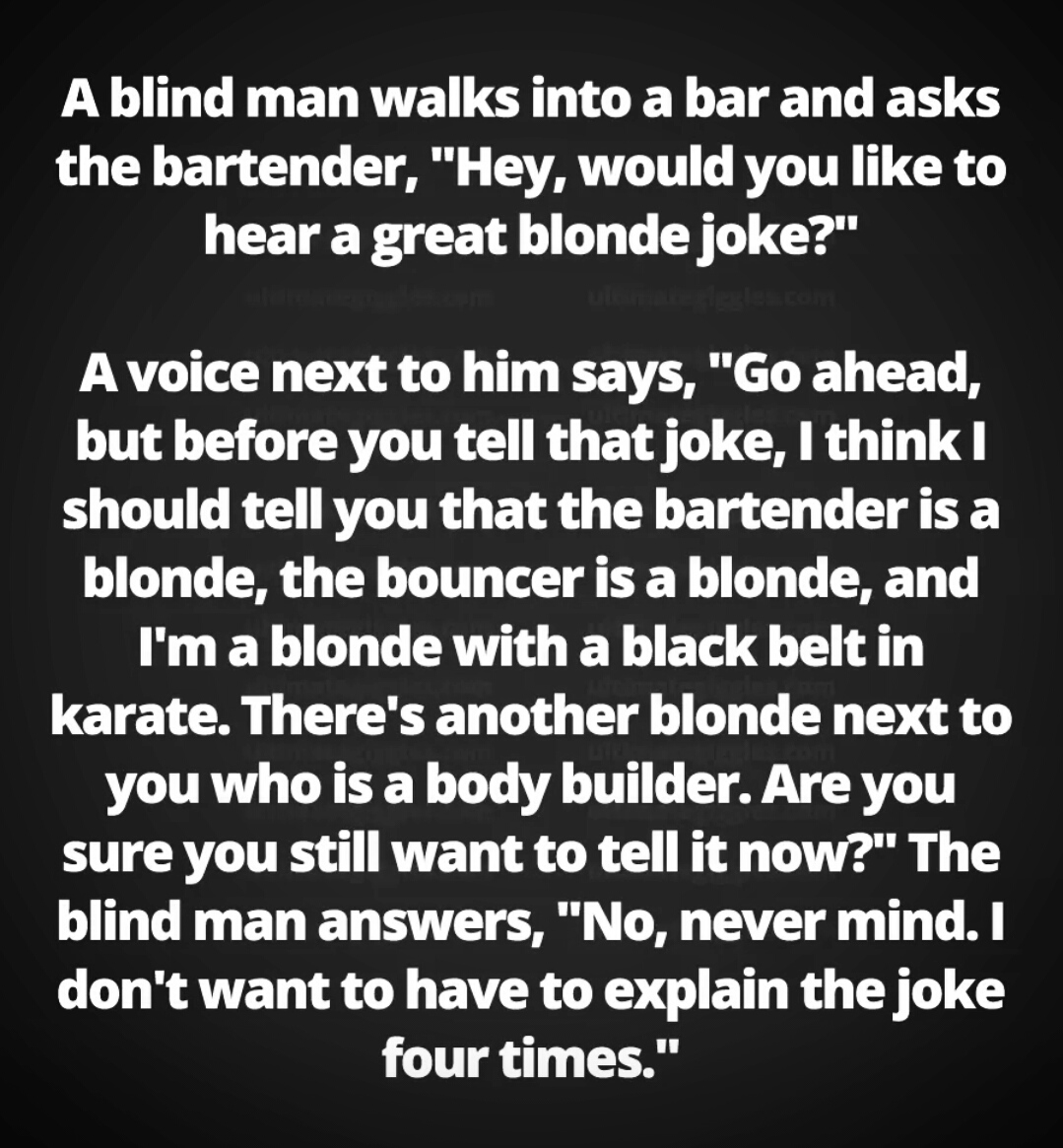The image features a humorous text-based joke displayed in bold white font on a solid black background, designed for social media sharing. The text is structured with a few lines at the top, followed by a break, and then the main content of the joke. The joke reads: "A blind man walks into a bar and asks the bartender, 'Hey, would you like to hear a great blonde joke?' A voice next to him says, 'Go ahead, but before you tell that joke, I should warn you that the bartender is a blonde, the bouncer is a blonde, and I'm a blonde with a black belt in karate. There's another blonde next to you who is a bodybuilder. Are you sure you still want to tell it now?' The blind man responds, 'No, never mind, I don't want to have to explain the joke four times.'" The text spans the width of the image with slight margins on either side, maintaining a clean and readable format.